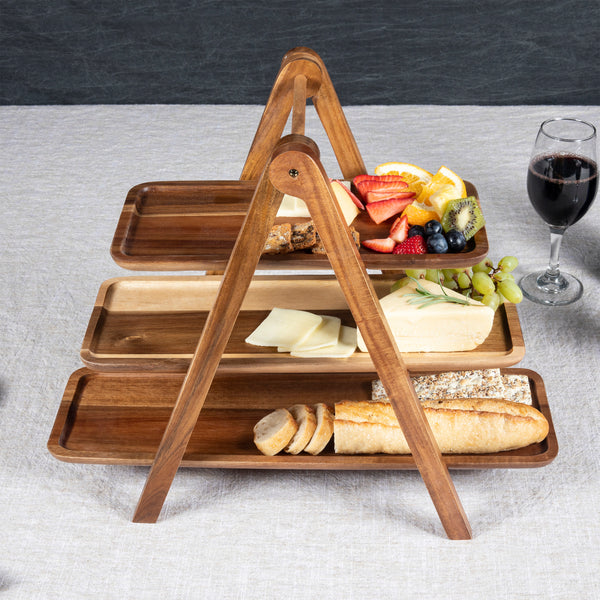This is a professionally styled photograph showcasing a creative charcuterie display set atop a wooden frame that resembles a swing set or easel. The frame is supported by two tripod legs spread outward on either end, with three wooden trays hanging vertically, one above the other. The arrangement is placed on a soft, white tablecloth with padding underneath, situated in front of a dark gray background. 

The bottom tray features a loaf of baguette with three slices cut off, accompanied by several long crackers. The middle tray displays a selection of cheeses, including a wedge of creamy brie and three slices of light yellow cheddar, alongside a bunch of fresh green grapes. The top tray is adorned with a vibrant assortment of fruits, such as orange slices, cut strawberries, kiwis, blueberries, and possibly apple slices. To the upper right of the setup, there is a glass of dark red wine, more than half full.

The arrangement of food items on each tray is predominantly to the right, and the entire setup exudes an air of elegance and freshness, enhanced by the soft, diffused lighting that casts subtle shadows in multiple directions.